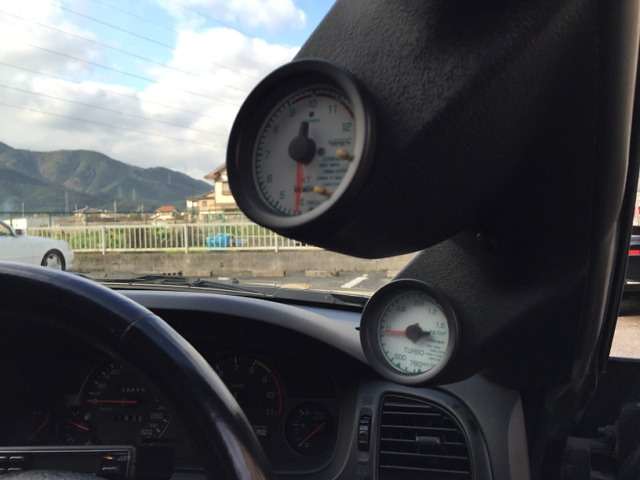This vivid color photograph captures the view from the driver's seat of a vehicle. The black steering wheel appears prominently in the lower left quadrant of the frame. The car's interior, also predominantly black, includes a centrally located air vent at the bottom of the image. Through the windshield, the outdoor scene displays a striking yellow metal fence juxtaposed against a backdrop of distant mountains.

A large gauge cluster, slightly out of focus, intrudes into the frame from the top right corner, extending towards the center. Composed of plastic and featuring dual humps, each hump houses a circular gauge. These gauges, characterized by white dials, black centers, and red needles, resemble clock faces. The upper gauge displays legible numbers, while the lower gauge is too blurred to discern.

The upper left portion of the image reveals a bright, cloudy sky intersected by telephone wires, adding to the complexity of the scene. The overall color palette of the photo is dominated by blacks and shades of white, with splashes of blue, green, and yellow from the external environment.